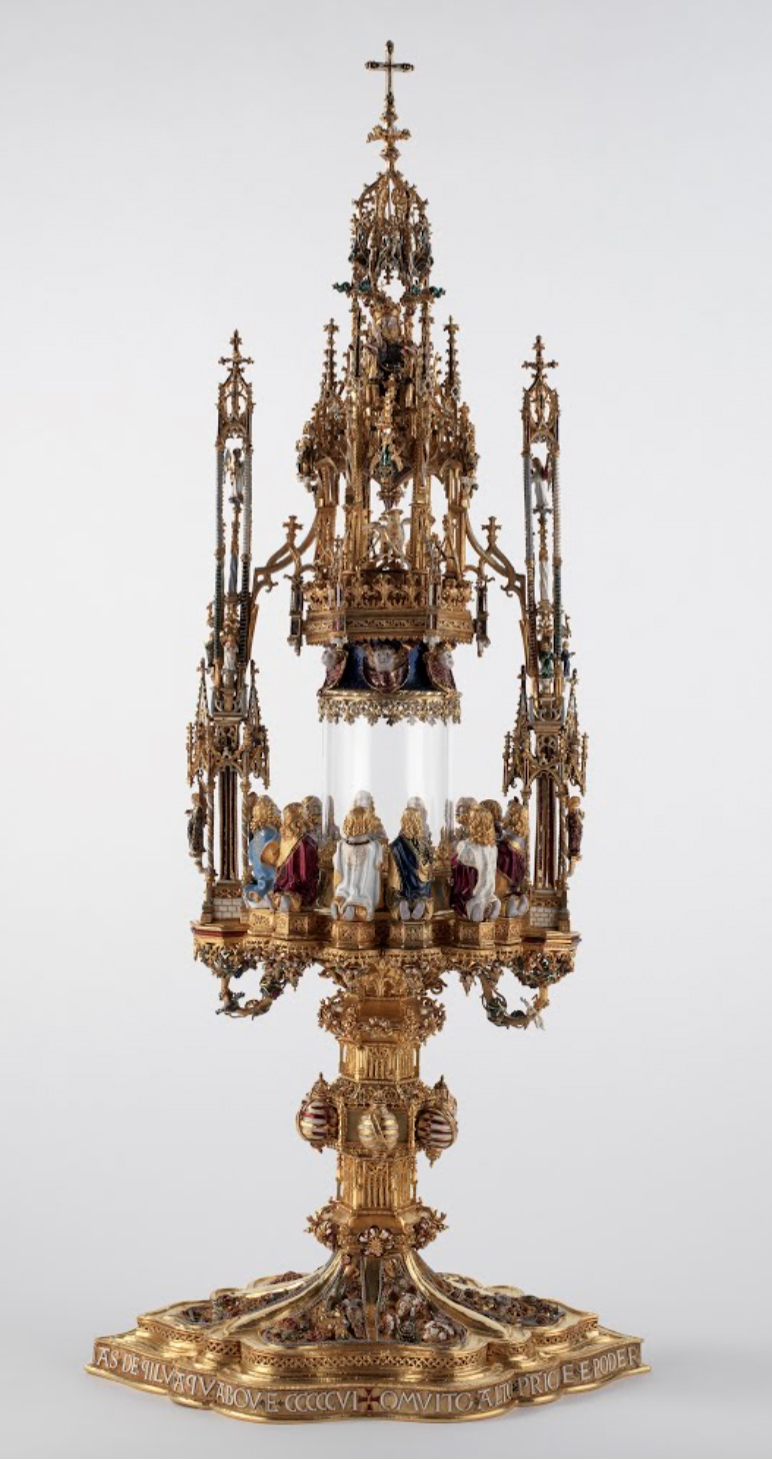This image portrays a substantial and ornate religious artifact, possibly from the Greek or Russian Orthodox tradition, set against a simple light gray backdrop. The piece is intricately designed, featuring elaborate metalwork that appears to be either brass or gold. It begins with a broad, decorative base that supports a pedestal adorned with complex decorations. Above the pedestal, a glass cylinder is centrally positioned, encircled by figures dressed in colorful, ornate robes—likely representing the Twelve Disciples. The structure ascends into multiple tiers, culminating in three spires each topped with a cross. The entire piece resembles a tree with ornaments or figures wrapped around its stem, combining elements of statue, art, and potentially functional aspects such as a candelabrum or a ceremonial lamp, minus any light source. Its complexity and religious iconography suggest it is a significant sacred object.